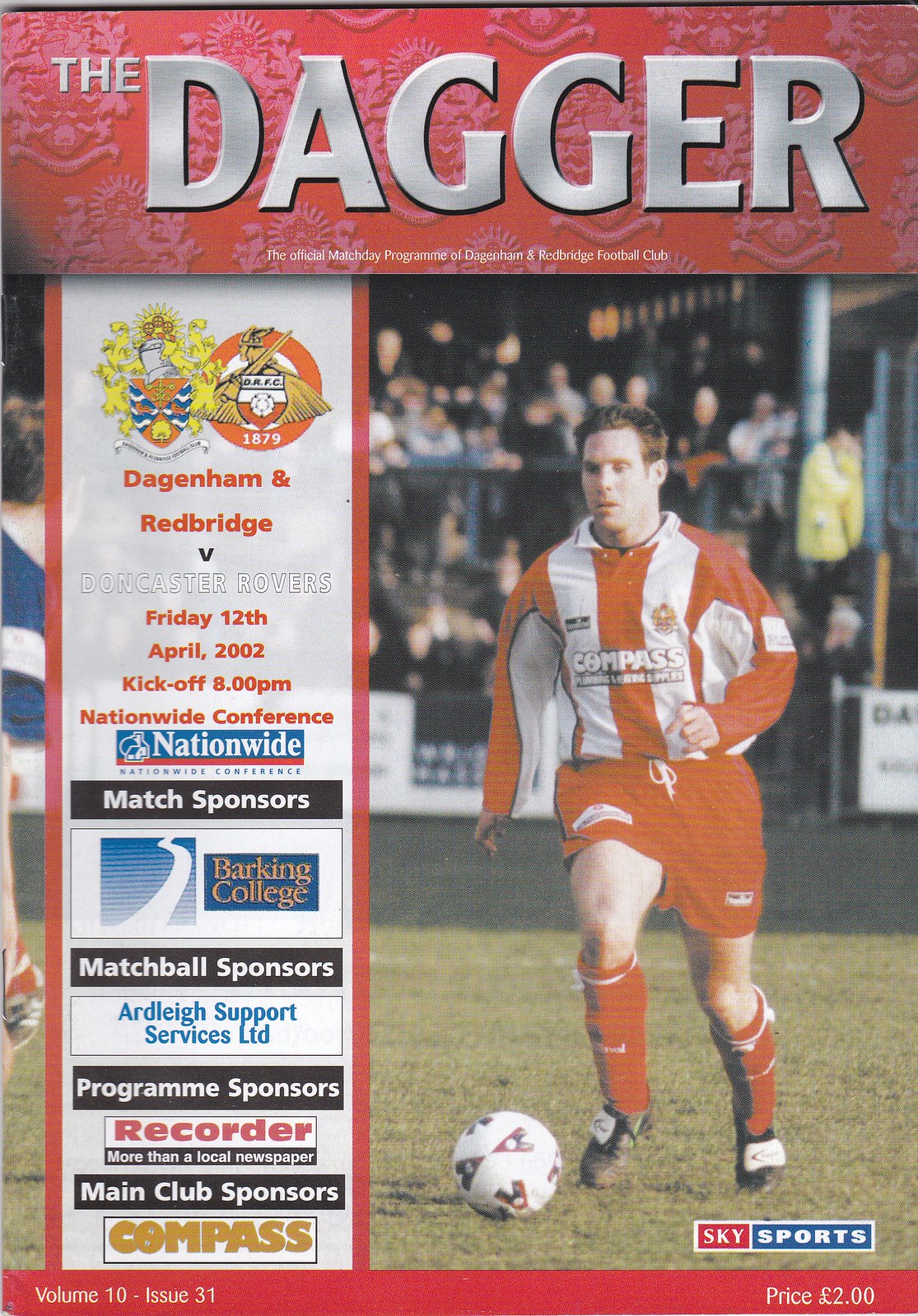The cover of the magazine titled "The Dagger" prominently features a single image of a soccer player in action. The player, a white male, is dribbling a soccer ball down the pitch. He is wearing an orange and white striped shirt, orange shorts, and orange socks, representing the team Compass. The upper portion of the cover displays the magazine's title in an embossed, metal-looking serif font over a repeating emblem pattern background. 

To the right of the photo, there are details about the soccer match between Dagenham Redbridge and Doncaster Rovers, scheduled for Friday, the 12th of April, 2002, with kickoff at 8 p.m. Below this information, a list of sponsors includes Nationwide, Barking College, Art Lace Board Program, Recorder, and Compass. The bottom right corner features the price of the magazine, set at 2 British pounds or 2 euros. Additionally, the lower side of the photo indicates Volume 10, Issue 31. The cover is filled with logos and icons of the sponsors and teams, while the background captures blurred spectators.